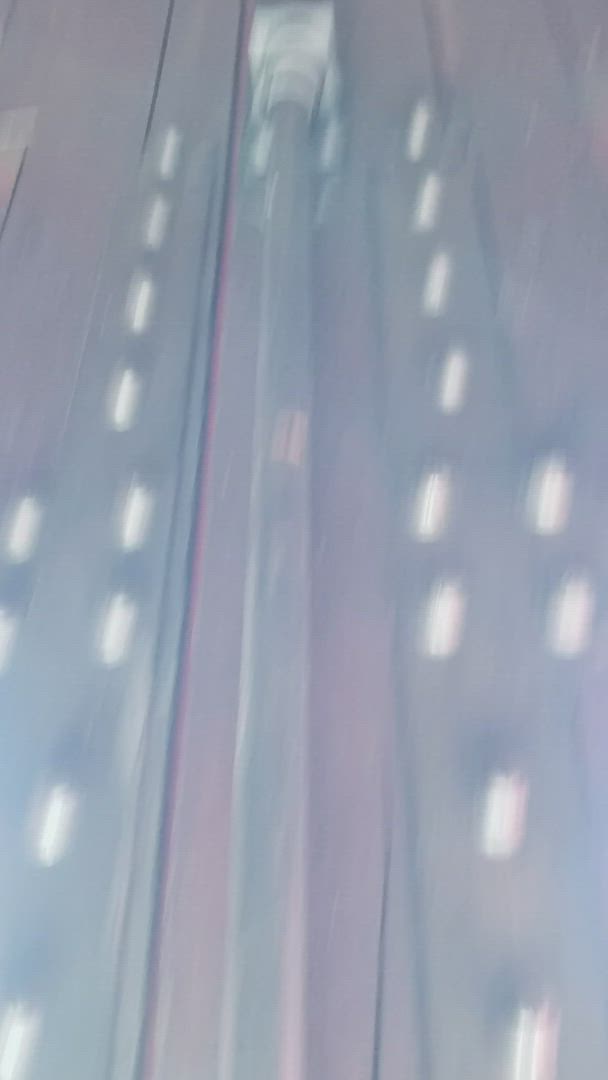The image is a blurry, close-up photograph of a vertical set-up that seems to depict some industrial or mechanical arrangement. In the center, there is a silver metal pipe that extends from the bottom and connects to a silver metal receptacle at the top, which has a rectangular structure on it. Flanking the pipe on both sides are black strips featuring small rivets at the top. The background has a purplish hue and appears to be composed of planks of wood, visibly showing cracks and different planks. Despite the blurriness, white dashes and possible tracks or trenches running vertically can be seen within the gray space surrounding the pipe, creating an impression of a racetrack, though the exact nature of the setup remains ambiguous.